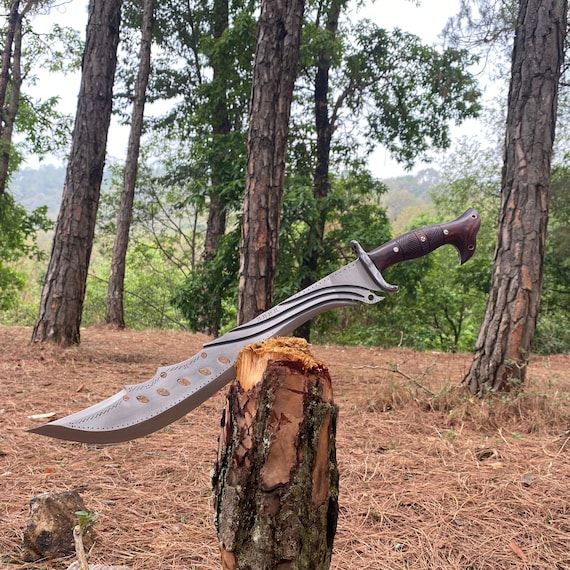In this image set in the wilderness, a large and intricately designed knife, described alternately as a machete, is prominently embedded at an angle into a roughly-hewn tree stump. The knife features a dark brown, curvy wooden handle with a pointed end, attached to a long, silver metallic blade. The blade's sharpened edge has a darker tint, with multiple rivets and wavy lines near its base, accentuating its sophisticated design.

The scene surrounding the stump and knife is a woodland area, covered with a thick layer of brown, dead pine needles and leaves, suggesting it is late in the season. In the immediate background, several tall, slender tree trunks, likely pine or evergreen, are visible. Beyond these, there are additional trees with lush green leaves, contrasted against a hazy, grayish-white sky that creates an overcast ambiance. The distant backdrop reveals a field with green brush, adding depth to the atmospheric forest setting. A smaller, older stump sits nearby, further adding to the rustic and untamed character of the landscape.